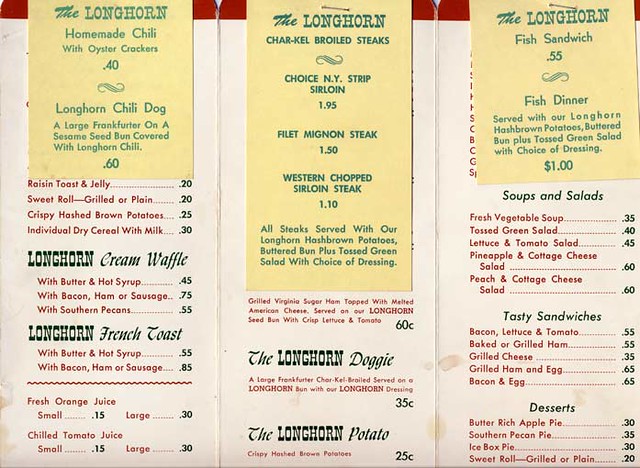This photograph captures an old-fashioned restaurant menu consisting of three panels with a mix of yellow-green and off-white backgrounds. 

### Top Panel
At the top of the menu, set against a faded yellowish background with green text, the following items are listed:

- **Homemade Chili with Oyster Crackers** - $0.40
- **Chili Dog** - A large Frankfurter on a sesame seed bun covered with Longhorn Chili - $0.60
- **Raisin Toast and Jelly** - $0.20
- **Sweet Roll, Grilled or Plain** - $0.20
- **Crispy Hashed Brown Potatoes** - $0.25
- **Individual Dace Dry Cereal with Milk** - $0.30
- **Cream Waffle** - $0.45 (with butter and hot syrup), $0.75 (with bacon, ham, or sausage), $0.55 (with Southern pecans)
- **French Toast** - $0.55 (with butter and hot syrup), $0.85 (with bacon, ham, or sausage)

Drink options with their prices are in red text with dark font prices:
- **Fresh Orange Juice** - Small $0.15, Large $0.30
- **Chilled Tomato Juice** - Small $0.15, Large $0.30

### Middle Panel
This section, primarily in a yellow background with green headers, lists various high-quality steak options:

- **Cracker Charcoal Broiled Steaks**
  - **Choice New York Strip Sirloin** - $1.95
  - **Filet Mignon Steak** - $1.50
  - **Western Chop Sirloin Steak** - $1.10

All steaks are served with Longhorn Hash Brown Potatoes, a buttered bun, and a tossed green salad with a choice of dressing. 

Other items:
- **Grilled Virginia Sugar Ham** - Topped with melted American cheese, served on a Longhorn seed bun with crisp lettuce and tomato - $0.60
- **The Longhorn Doggy** - A large charbroiled shredded beef patty served on a Longhorn bun with Longhorn dressing - $0.35
- **The Longhorn Potato** - Crispy hash brown potatoes - $0.25

### Bottom Panel
The final panel with a green font heading and off-white background lists fish, soups, salads, sandwiches, and desserts.

- **Fish Sandwich** - $0.55
- **Fish Dinner** - Served with Longhorn Hash Brown Potatoes, buttered bun, and tossed green salad with choice of dressing - $1.00
- **Soups and Salads**
  - **Fresh Vegetable Soup** - $0.35
  - **Tossed Green Salad** - $0.40
  - **Lettuce and Tomato Salad** - $0.45
  - **Pineapple and Cottage Cheese Salad** - $0.60
  - **Peach and Cottage Cheese Salad** - $0.60

- **Tasty Sandwiches**
  - **Bacon, Lettuce, and Tomato** - $0.55
  - **Baked or Grilled Ham** - $0.55
  - **Grilled Cheese** - $0.35
  - **Grilled Ham and Egg** - $0.65
  - **Bacon and Egg** - $0.65

- **Desserts**
  - **Butter Rich Apple Pie** - $0.30
  - **Southern Pecan Pie** - $0.35
  - **Ice Box Pie** - $0.30
  - **Sweet Roll, Grilled or Plain** - $0.20

This detailed menu showcases a variety of homestyle American dishes and beverages, capturing the charm and simplicity of a bygone era.